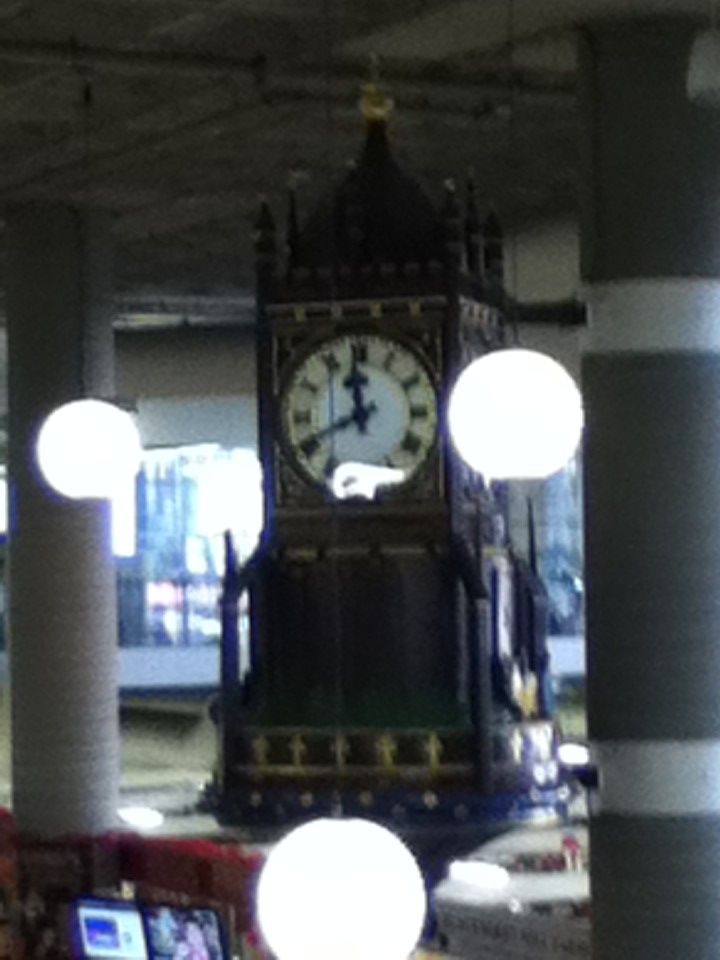This is a blurry color photograph capturing a tall structure resembling a clock tower. The clock, housed within an ornate, spired casing, features a beige and white face adorned with Roman numerals for the hours. Elegantly designed, the black hands of the clock point to approximately 11:40. Flanking the tower are glowing white globe lights, which add an ambient touch to the scene. At the bottom left corner, a computer monitor is partially visible. Notably, the vertical orientation of the image accentuates the tower's height. The photograph is devoid of people, animals, birds, or any text.